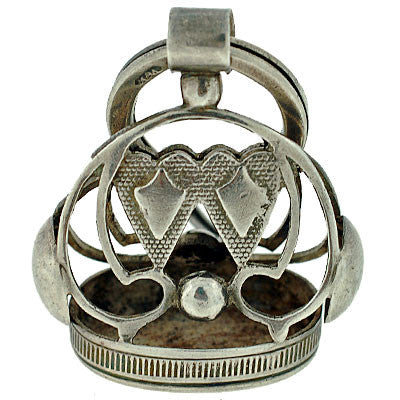The image features a unique, antique-looking metal object against a plain white background. The primarily silver device, accented with shades of brown, boasts a circular base adorned with numerous openings—approximately 60 to 70—creating an ornate and intricate design. It is reminiscent of a crown, with two prominent heart shapes at its center, each containing a diamond-like pattern. Below these hearts is a textured gold 'W' and surrounding apostrophe-shaped metal bars. The object is partially welded together, with some parts featuring a rough texture. At the top, a ring-like structure suggests it might be intended as a pendant or decorative piece, though its exact use is unclear.